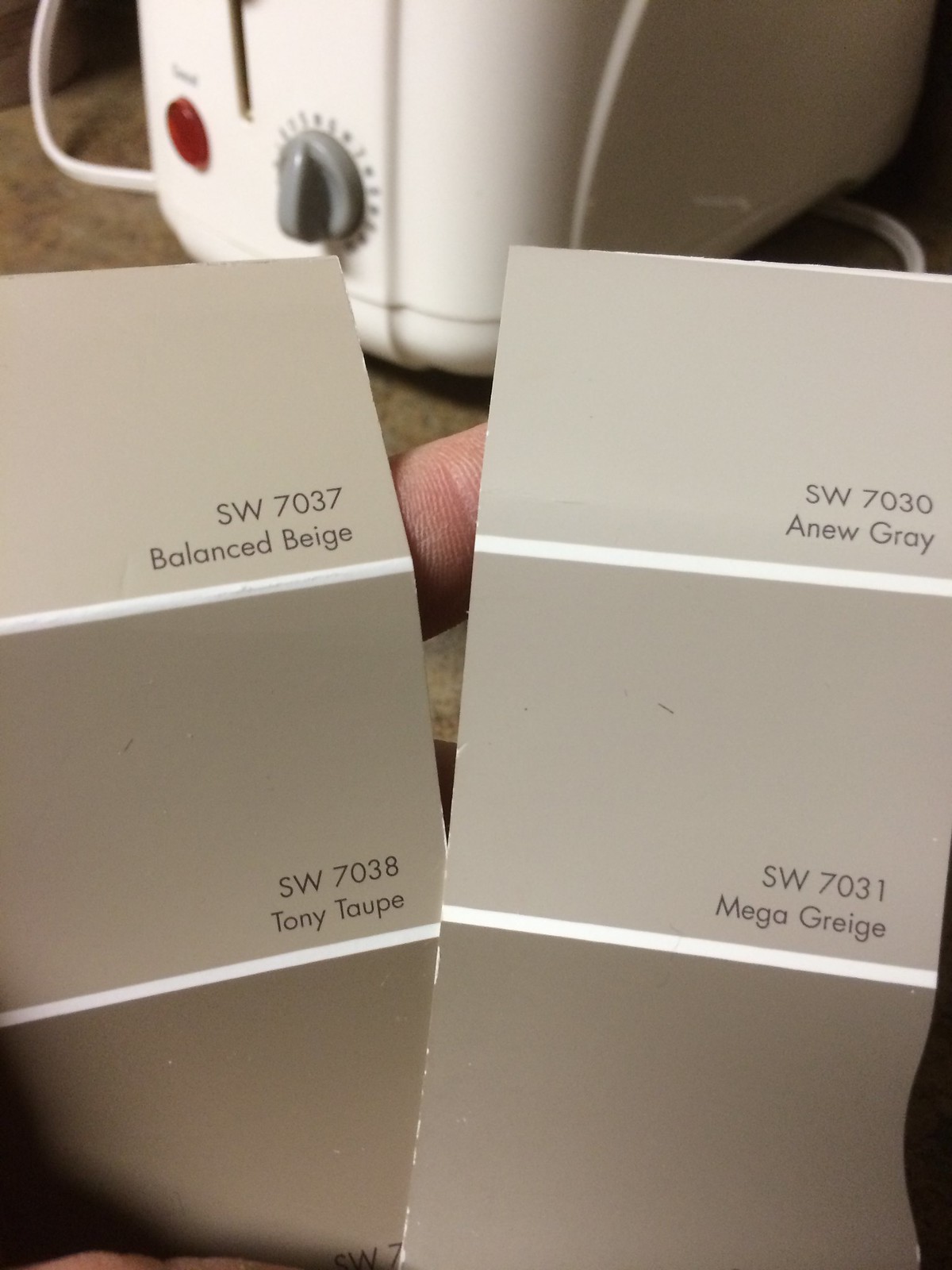The photograph captures a close-up of a hand holding two color swatch strips, each displaying three different paint shades. The first strip features SW7037 Balanced Beige, SW7038 Tony Taupe, and a third color partially obscured by the finger. The second strip displays SW7030 A New Gray, SW7031 Mega Graysh, and another unseen color. Each swatch is separated by thin white lines. In the background, a white kitchen appliance, possibly a toaster, sits on a countertop, indicating that the person is likely selecting paint colors for a kitchen renovation. The swatches show subtly varying hues of beige and gray, showcasing different options for potential color schemes.